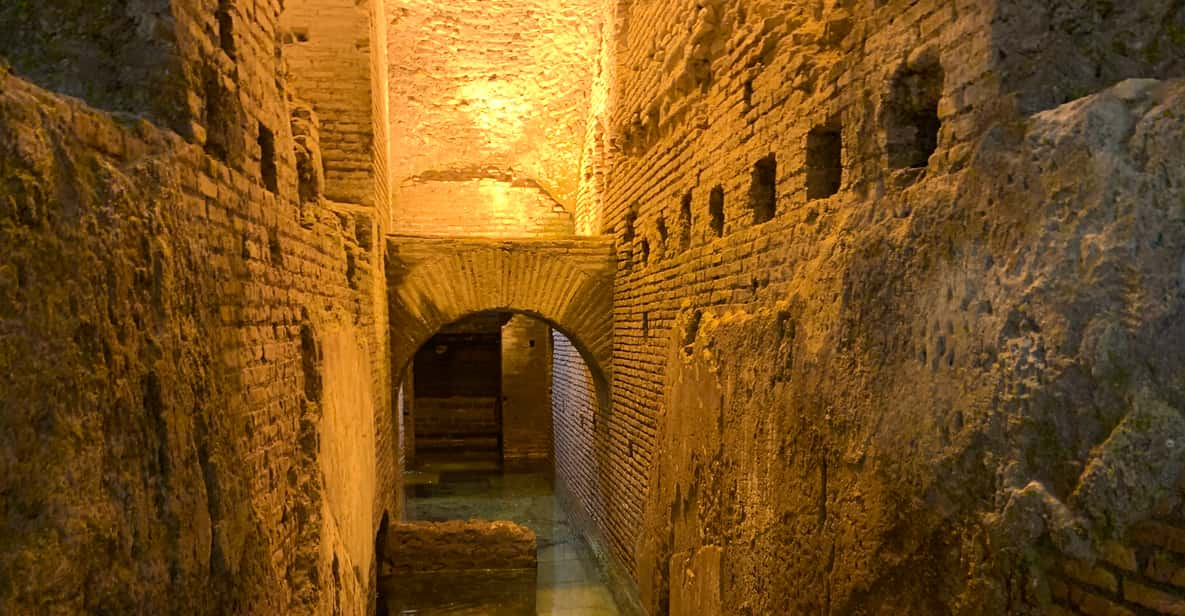This photograph depicts the partial ruins of an ancient structure, possibly a temple, sewer, or canal, characterized by its heavily weathered and crumbling stone and brickwork. The walls, composed of uniformly stacked bricks that exhibit a warm palette of tan, beige, orangish-brown, and yellow hues, are partially exposed with some sections covered in a rough, concrete-like polymer, enhancing the sense of antiquity and fragility. Central to the image is an archway leading down a dim hallway, with a faint light source illuminating the end. The floor under the archway appears to be layered with a shallow pool of water, adding a greenish-gray tint to the scene. This interplay of light and shadow accentuates the broken, uneven texture of the brickwork, conveying a deeply evocative sense of age and history.